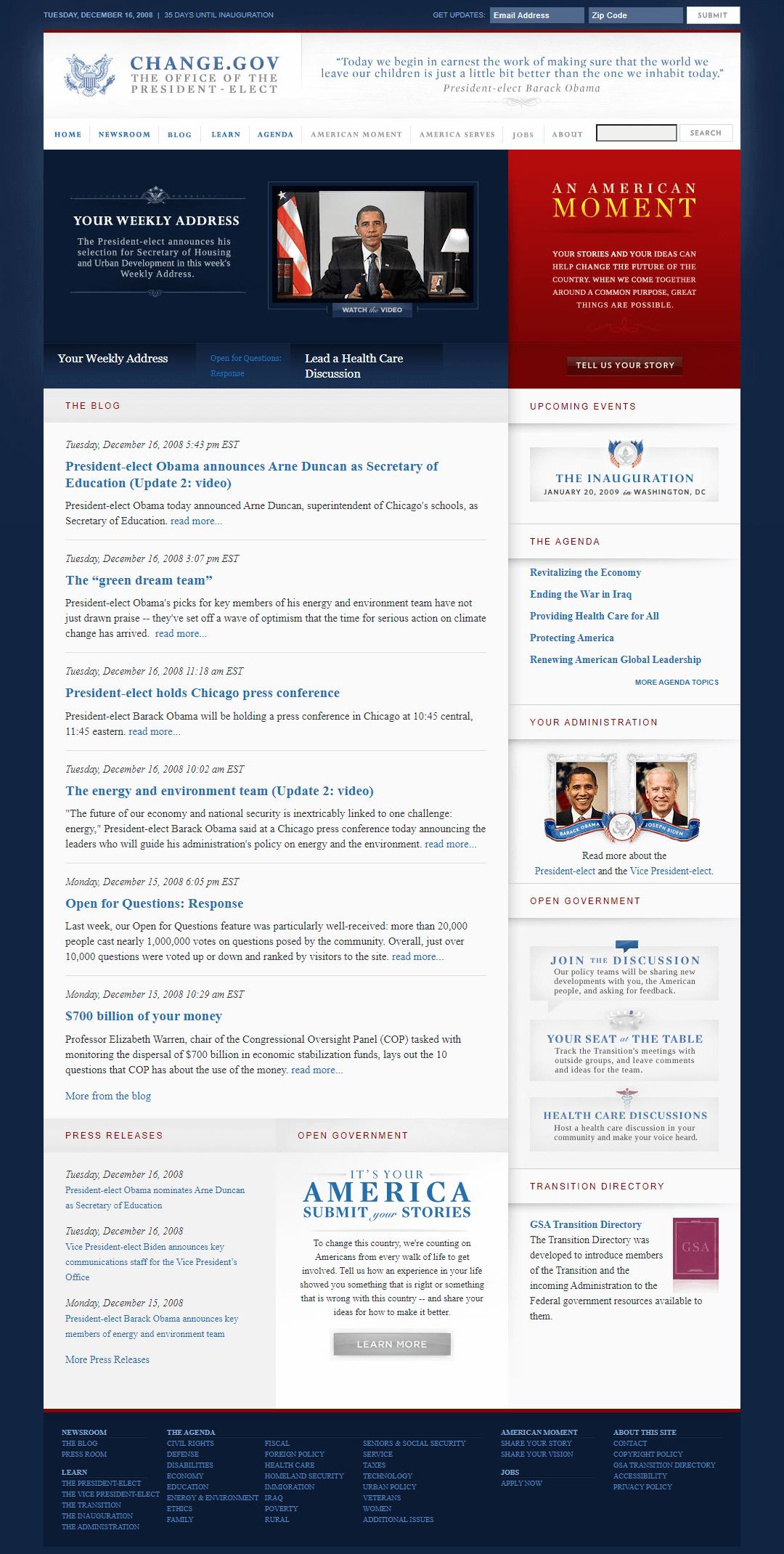This is a screenshot of the website "change.gov." The site’s name, "change.gov," is displayed in blue text, with the phrase "The Office of the President-Elect" written in black text directly underneath. To the left of this text is a logo, possibly the presidential seal. Below this header, the background transitions to a dark blue and features a small, centered image of a man, likely Barack Obama, though the image is too small to confirm definitively. 

To the left of the picture, the text reads "Your Weekly Address." To the right, within a red square, the phrase "An American Moment" appears in yellow text. 

Further down, there are various subject headings in blue text under a section labeled "The Blog" in red text. Each subject heading is followed by several lines of black text providing descriptions. At the bottom, a call to action in blue text states, "It's Your America," followed by "Submit Your Stories."

To the right of these subject matters is a column with headings such as "The Inauguration" and "The Agenda." Below these headings, images of two men—presumably Barack Obama on the left and Joe Biden on the right—are displayed under the title "Your Administration." Additional text in this column features subjects in blue, with their corresponding descriptions in black text.